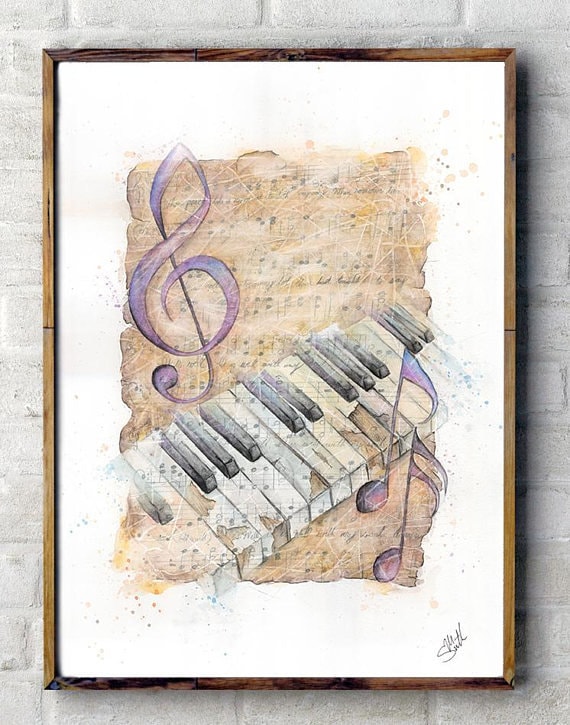This is a photograph of a framed piece of art hanging on a gray brick wall. The elegant frame is a mix of light oak and walnut tones, complemented with a decorative gold or bronze trim. The artwork within, set against a white background with scattered color spots, showcases a section of piano keys, both black and white. These keys, numbering about fifteen, are marked with a gentle brown patina, giving them a vintage look. Behind the keys is a vertically oriented sheet of tan-brown music paper. Prominently displayed on this sheet are various musical notes in purple, with a notable clef sign. The piece is signed at the bottom by the artist, Mr. Smith, creating a harmonious blend of neutral hues highlighted with subtle purple accents, perfect for a music-themed room.